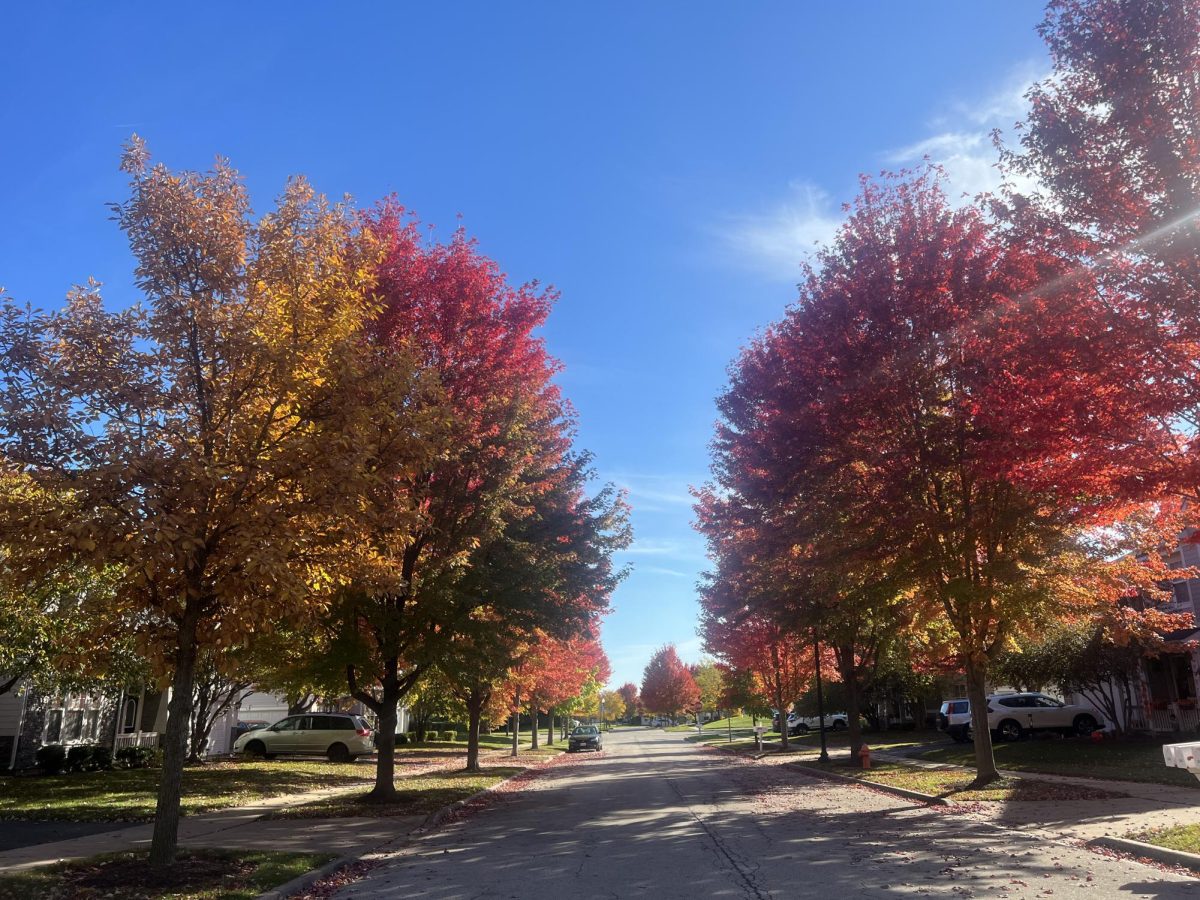This color photograph captures a picturesque residential street on a sunny, clear autumn afternoon, possibly in a small town in the Northeastern United States. The scene is defined by a blue sky with wispy, powdery clouds. Both sides of the paved asphalt road are lined with large maple trees exhibiting a stunning array of fall colors, from vibrant yellow and red to shades of orange and green. Fallen leaves scatter across the sidewalks. Several cars, including minivans and SUVs, are parked along the street and in driveways. Notably, there's a white house with a garage and a van parked in front of it. The neighborhood features typical suburban houses, mostly one story with attics, partially obscured by the colorful foliage. The overall impression is one of serene suburban charm in the heart of autumn.